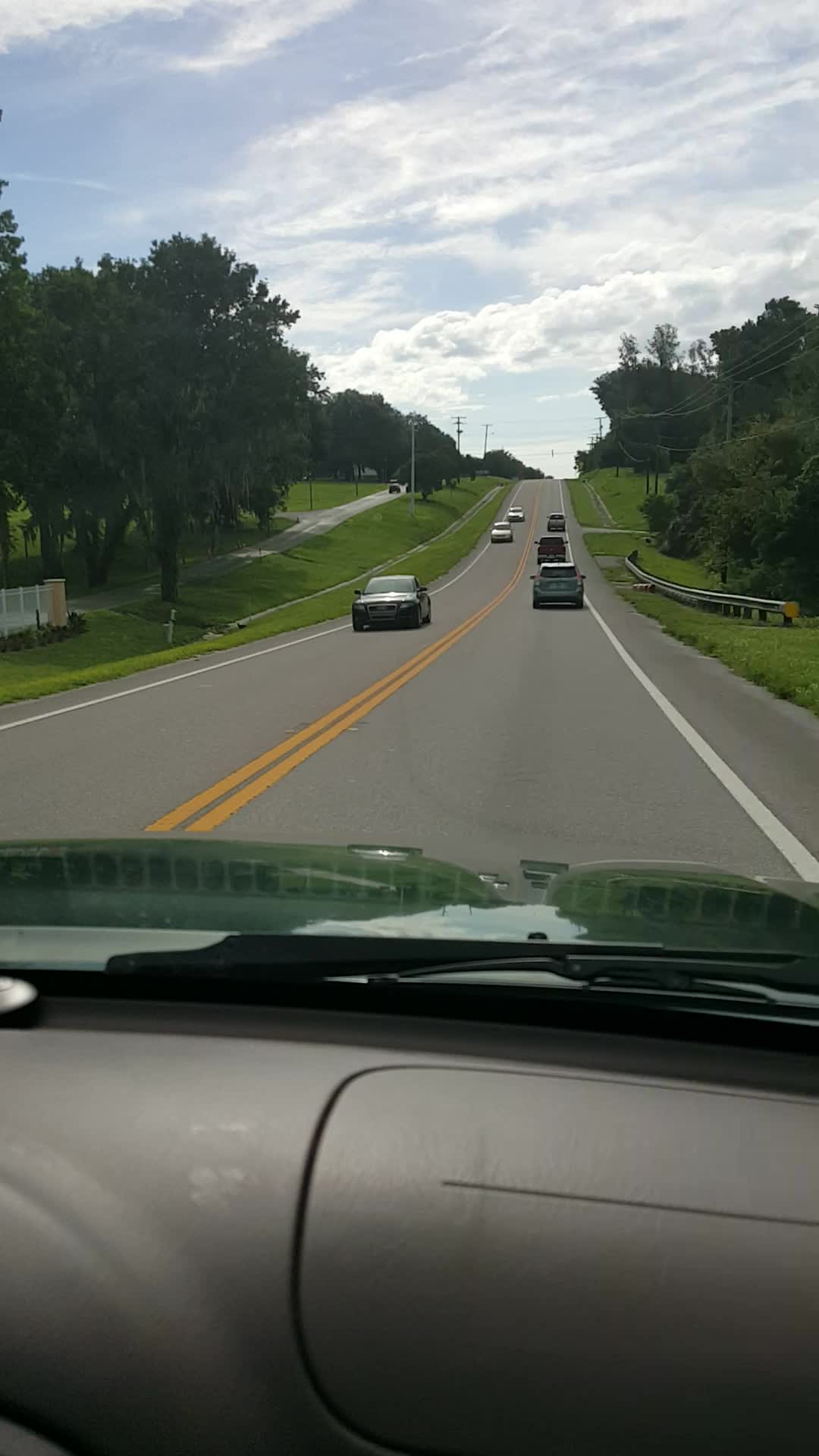A vibrant color photograph captures a scene from inside a vehicle, taken through the windshield. The gray dashboard is partially visible at the bottom of the image, along with a windshield wiper on the right and reflections on the glass. Ahead lies a long, black road that curves gently towards the horizon, bordered by a double yellow line. Three cars are visible in the lane ahead, moving away from the viewer, while three other cars travel in the opposite direction towards the viewer. 

To the right, there is a grassy area flanked by a metal guardrail, featuring several tall trees, telephone poles, and wires. The left side mirrors this setup, with a green lawn, a narrow sidewalk, and what seems to be a park adorned with tall trees. The overcast sky adds a muted, contemplative atmosphere to the scene. The image, taller than it is wide, encapsulates a fleeting moment on a typical roadway, framed by nature and utility.